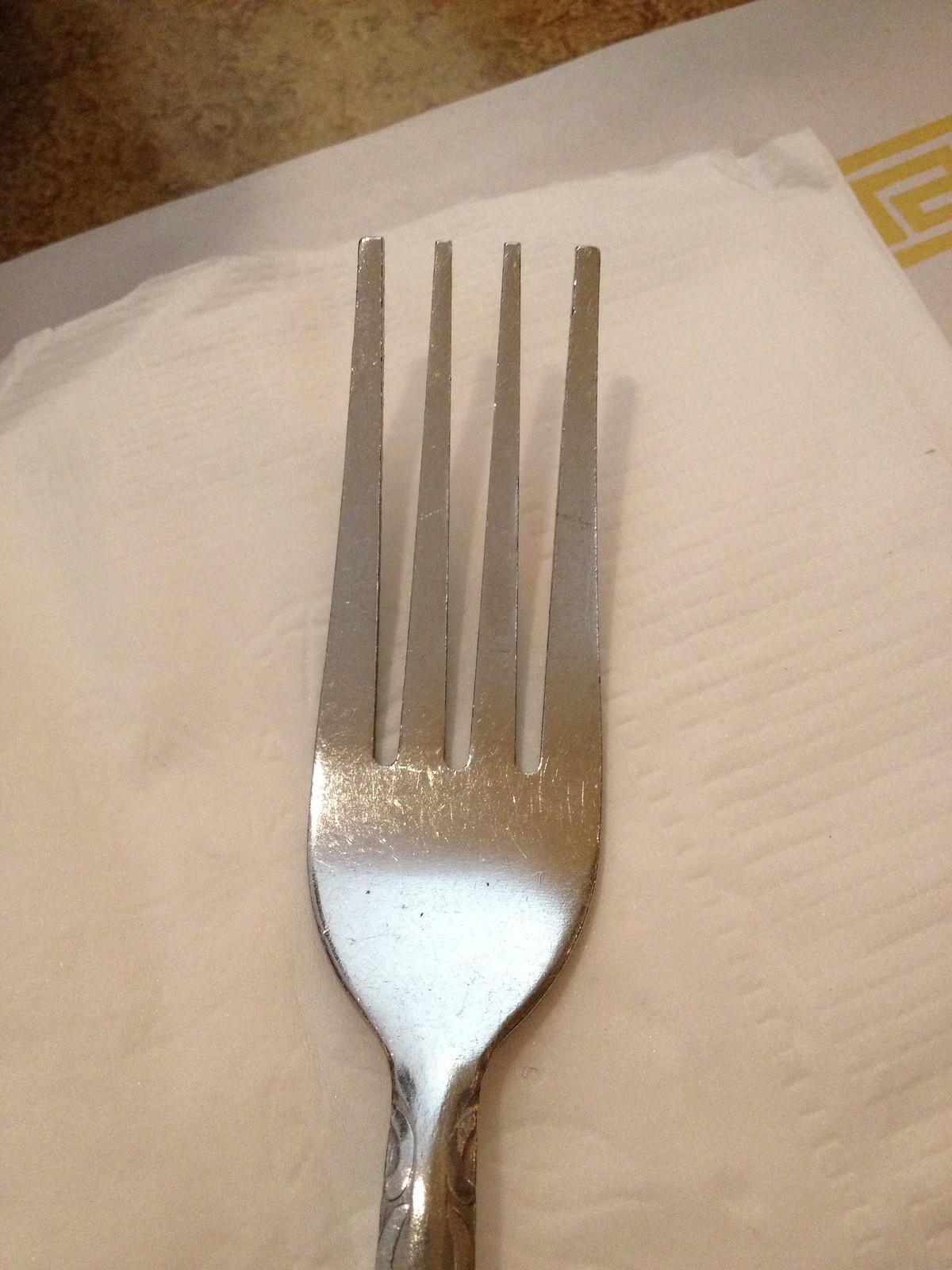In this photograph, we see an extreme close-up of a slightly scratched silver chrome fork, captured in a restaurant setting. The image focuses on the upper part of the fork, revealing four slightly blunt prongs and a subtly textured neck with a faint floral motif. The fork rests on a plain white napkin, which is embossed with light imprints, possibly floral in nature. This napkin covers part of a decorated white plate, showcasing a simple, geometric, square pattern at the top right corner that evokes Chinese design elements. The background reveals a white paper placemat with a small gold symbol, possibly indicative of a Greek or Chinese restaurant, resting on a brown and beige table. The setting is minimal yet carefully detailed, with no visible text or writing.